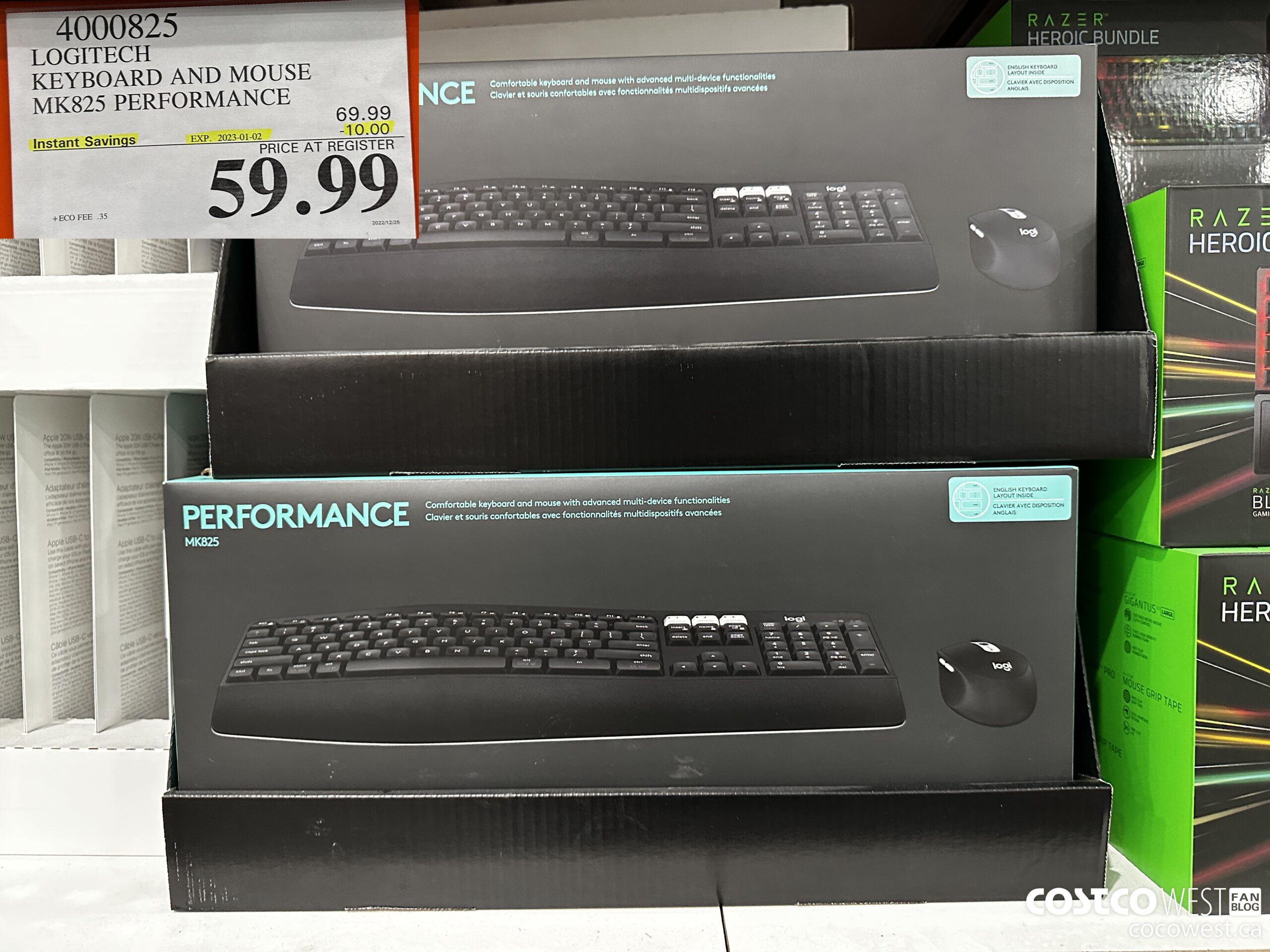The photograph captures a retail display of products on a store shelf, prominently featuring a Logitech keyboard and mouse set.

At the top left of the image, a hanging tag is visible. The tag features a white piece of paper with red lines on the left and right edges. At the top left of the tag, black numbers read "400825." Below this, there are three lines of black text in all caps stating, "LOGITECH KEYBOARD AND MOUSE," followed by "MK825 PERFORMANCE." 

Further down to the right, the large black numeral "69.99" is displayed, indicating the price before any discounts. Below this numeral, there is a row of highlighted information. The first section, highlighted in black, reads "INSTANT SAVINGS." The middle section, which is smaller in size, notes "EXP. 2023-01-02," specifying the expiration date of the offer. The final section underneath "69.99" shows "-10.00," indicating a ten-dollar discount. A black line separates this information from the next section.

On the right side of the tag, additional black all-caps text states "PRICE AT REGISTER." This is followed by bold, large black numerals displaying the discounted price of "59.99."

Below the tag and to the right, the shelf displays boxes of keyboards. These boxes feature a dark gray background and display an image of an ergonomic keyboard, accompanied by a black mouse positioned to the right. In the top left corner of these boxes, light blue text reads "PERFORMANCE." The top right corner of the boxes contains a light blue rectangle with black text on it. These product boxes are nested within black display boxes.

To the right of the Logitech products, there are boxes of other items on the shelf. These boxes have a green left side, a black front, and are adorned with multicolored lines. At the bottom right of the photograph, an overlay with white text reads "COSTCO WEST," indicating the location or store name.

The scene is set against the backdrop of a typical retail environment, displaying a well-organized and detailed presentation of the products available for purchase.